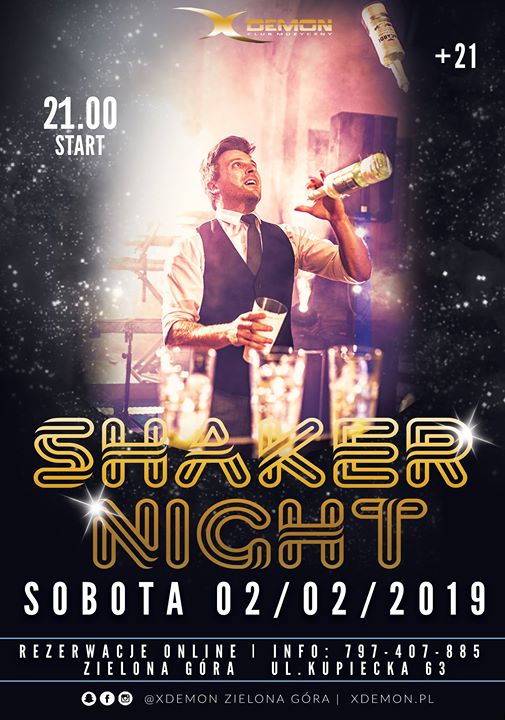The image is a digitally created poster for a nightclub event titled "Shaker Night," scheduled for February 2, 2019. Dominating the poster is an animated male bartender, skillfully mixing drinks with a cocktail shaker and bottle, suggesting a flair bartending performance. He is positioned towards the left, gazing upwards to the top right, with his bent arm holding the bottle. The text, primarily in gold, white, and black, includes details such as "Demon," "21 Start," "Plus 21," and "Sobota 2-2-2019," distributed across the top and bottom of the image. The background features a palette of black, white, gray, gold, yellow, red, and purple, creating a vibrant nightlife atmosphere. The objects and text are well-spaced, contributing to a clear and engaging design intended to advertise the lively nightclub event.